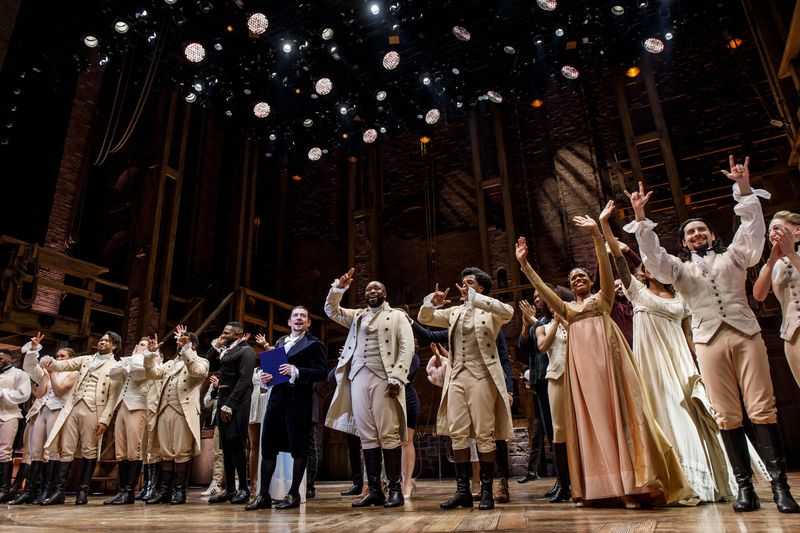The image showcases a theatrical performance, likely a scene from the play "Hamilton." The stage, with its wooden structure and hardwood floor, is filled with actors dressed in ornate 16th or 17th-century attire. The men are predominantly wearing vests, many of which are white in the middle, and some have velvety black and blue suits. One notable man with a velvety suit holds a blue book and stands next to another in a black suit. Their attire includes tall black boots, soft fabric pants tucked into the boots, pointed buttoned vests, blousey shirts with ruffled collars and sleeves, or jackets with coattails. Among them, women don pink and white gowns. The scene suggests the conclusion of a performance as the cast makes signs and waves to the audience. Above, around 50 colorful spotlights illuminate the stage, and bubbles descend from the ceiling, adding a festive touch to the atmosphere.